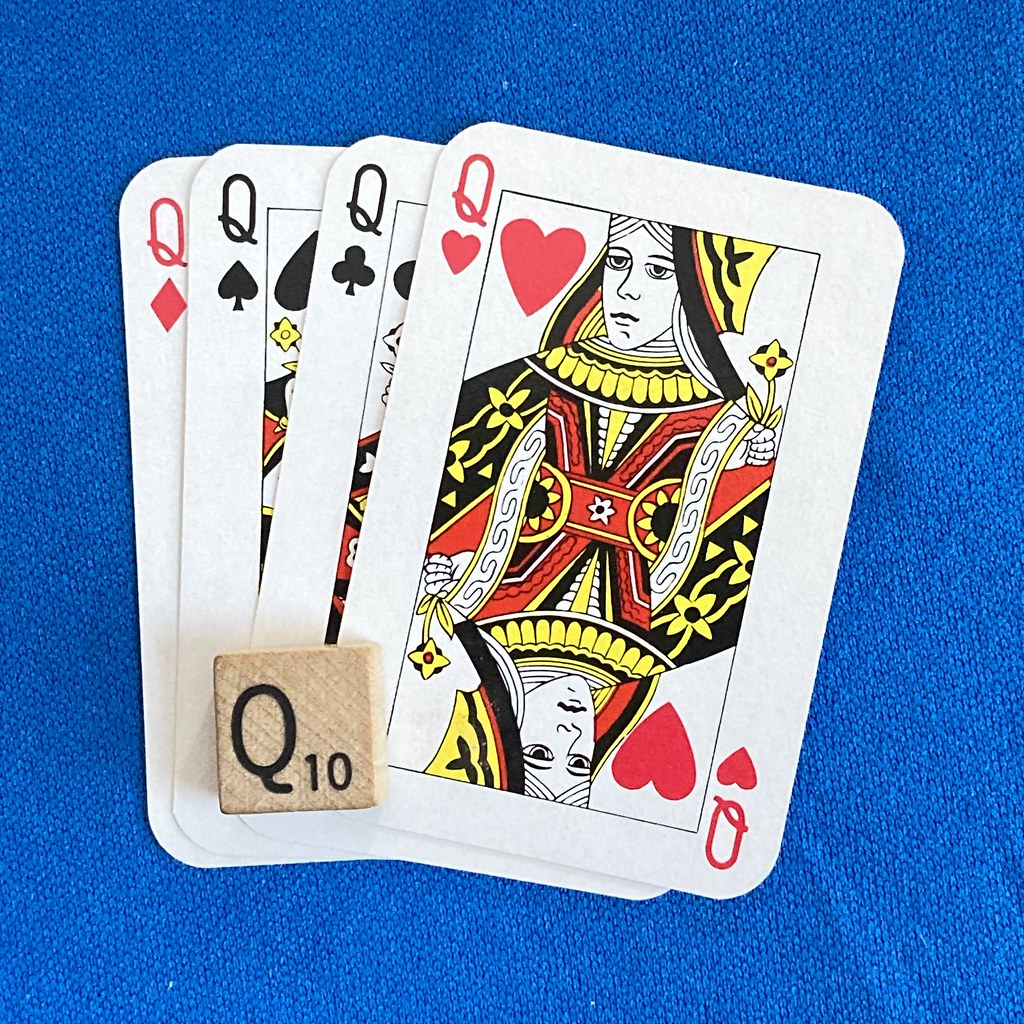A close-up image showcases a set of playing cards meticulously arranged on a vibrant blue fabric backdrop. The focal point of the composition is the Queen of Hearts card, prominently displayed at the top of the ensemble. Beneath it, partially obscured, lies the Queen of Clubs, followed by the Queen of Spades, and finally, the Queen of Diamonds, with only its "Q" and diamond symbol subtly visible. Atop this regal assembly rests a single Scrabble tile, the letter "Q" marked with a value of 10 points, adding a whimsical touch. The playing cards, part of a standard deck, and the wooden Scrabble tile are both ordinary in design, emphasizing simplicity. Together, the arrangement underscores a thematic celebration of the letter "Q," unified in an elegant, zoomed-in display.